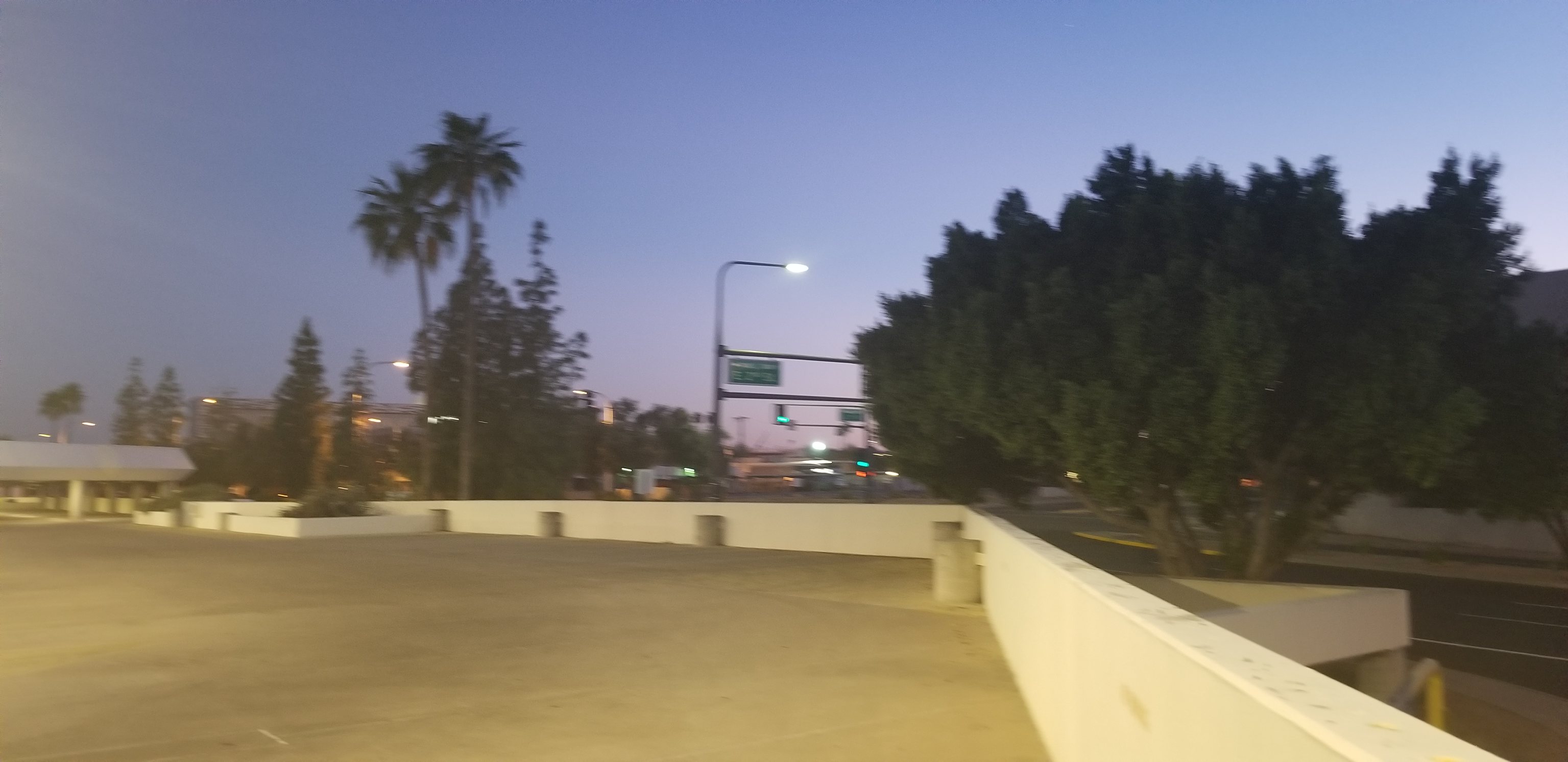The image depicts a scenic view from a rooftop parking lot at sunset, with a purplish tint to the evening sky. The foreground features a concrete walkway extending from the left side center, leading down to the bottom of the image. A concrete barrier runs along the edge of the walkway, accompanied by potted plants. To the far left, a white awning is held up by a single pillar, resembling a sculpture. Further in the distance to the left, a tall palm tree stands prominently, with additional conifer trees and a light pole with illuminated signage nearby. Nestled amidst these elements is a large green bush. The background showcases a road, possibly a freeway exit, which is barely visible along with several stoplights. A large brown building can be seen faintly in the far distance. The scene is complemented by a serene tree line framing the sky, enhancing the tranquil, twilight ambiance.